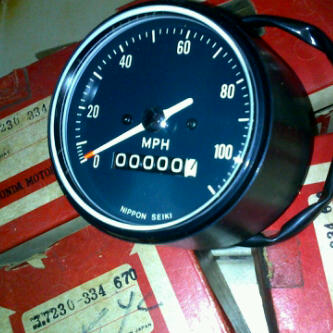The image displays a classic, standalone speedometer with its needle fixed at 0, and the odometer reading 00000.7. The odometer digits are predominantly black except for the tenths place, which is in white. The speedometer is calibrated up to 120 mph, with major increments marked at every 20 mph (0, 20, 40, 60, 80, 100, 120) and minor lines indicating the numbers in between. The device is not installed in a vehicle but is instead resting on several old, worn cardboard boxes, which appear to be deeply etched and printed with dark numbers. One of the boxes is marked in black marker, showing the letters "NYC" or "YC." The red color of the boxes is significantly faded in several areas. The speedometer itself features a shiny black body, housing a black face with white numerals, and a possible handle or covered wire extending from the top to the bottom.